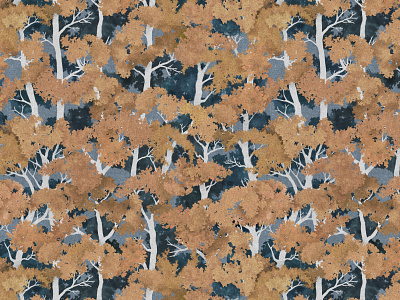The image features a detailed, colour-filled artwork that spans the entire frame in a landscape orientation. The medium is indeterminate, possibly digitally rendered, and showcases a close-up shot of what appears to be trees or bushes, creating an impression of a dense, forested area. The foliage is depicted in varied shades of brown, ranging from lighter to darker hues. White trunks or branches are visible in the gaps between the clusters of leaves or flowers, contributing to the overall texture.

The artwork has an abstract quality and appears to be a repeating tile pattern, forming a seamless image that extends across the canvas. The background consists of darker blues and grays, which might represent more foliage or the forest in shadow, adding a sense of depth and mystery. The overall color palette includes light and dark gray, white, and an assortment of brown tones, evoking an autumnal atmosphere.

The trees, possibly resembling aspens or birches due to their white trunks, have their brown leaves clustered rather than individually detailed. The painting gives the impression of looking either upwards at the tree canopies or a bird's-eye perspective. Some branches extend from the trunks, ending in bare twigs. This repetitive, pattern-like nature of the composition creates a uniform yet immersive visual experience, making it difficult to discern the scale or height of the trees, enhancing its abstract and potentially meditative quality.